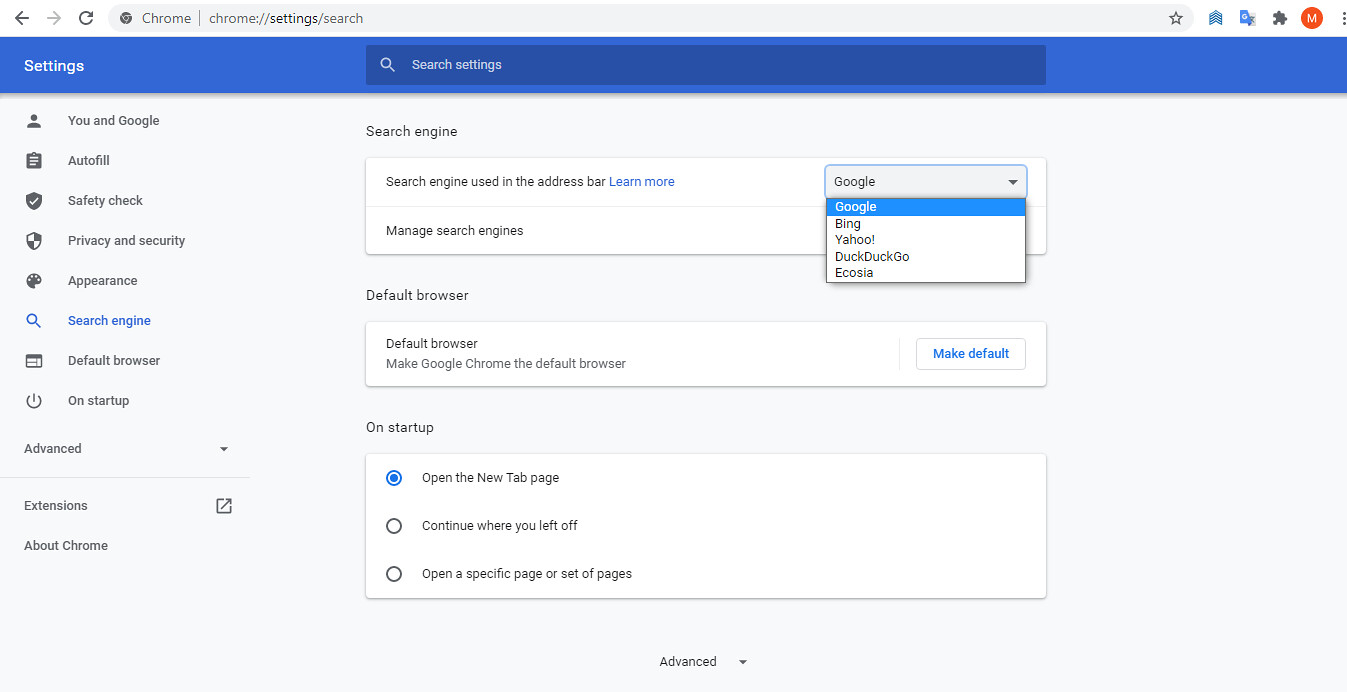This image is a detailed screenshot of a Chrome browser window on a desktop or laptop PC. In the upper left corner, the browser's navigation arrows for going back and forth are visible, followed by the refresh button. Adjacent to these is the address bar, displaying the text "Chrome, Chrome, Settings Search". To the right of the address bar, several icons represent various installed add-ons.

The main window features a blue bar at the top indicating the "Settings" page, with a search bar positioned to the left-hand side. The left sidebar menu includes categories such as "You and Google," "Autofill," "Safety Check," "Privacy and Security," "Appearance," "Search Engine," "Default Browser," "On Startup," and options for "Advanced," "Extensions," and "About Chrome."

In the central part of the page, a section labeled "Search Engine" is displayed. Within it is a white box containing the text "Search Engine used in the address bar" with a "Learn More" link and a drop-down menu for selecting different search engines. Additionally, the section includes an option labeled "Manage Search Engines."

Below the "Search Engine" section is a "Default Browser" section, where a white box reads "Make Google Chrome the default browser." To the right of this text, a light blue button labeled "Make Default" is present.

Further down, a section titled "On Startup" appears, featuring three radio buttons with options: "Open the New Tab page," "Continue where you left off," and "Open a specific page or set of pages." At the very bottom of the page, there is a drop-down labeled "Advanced."